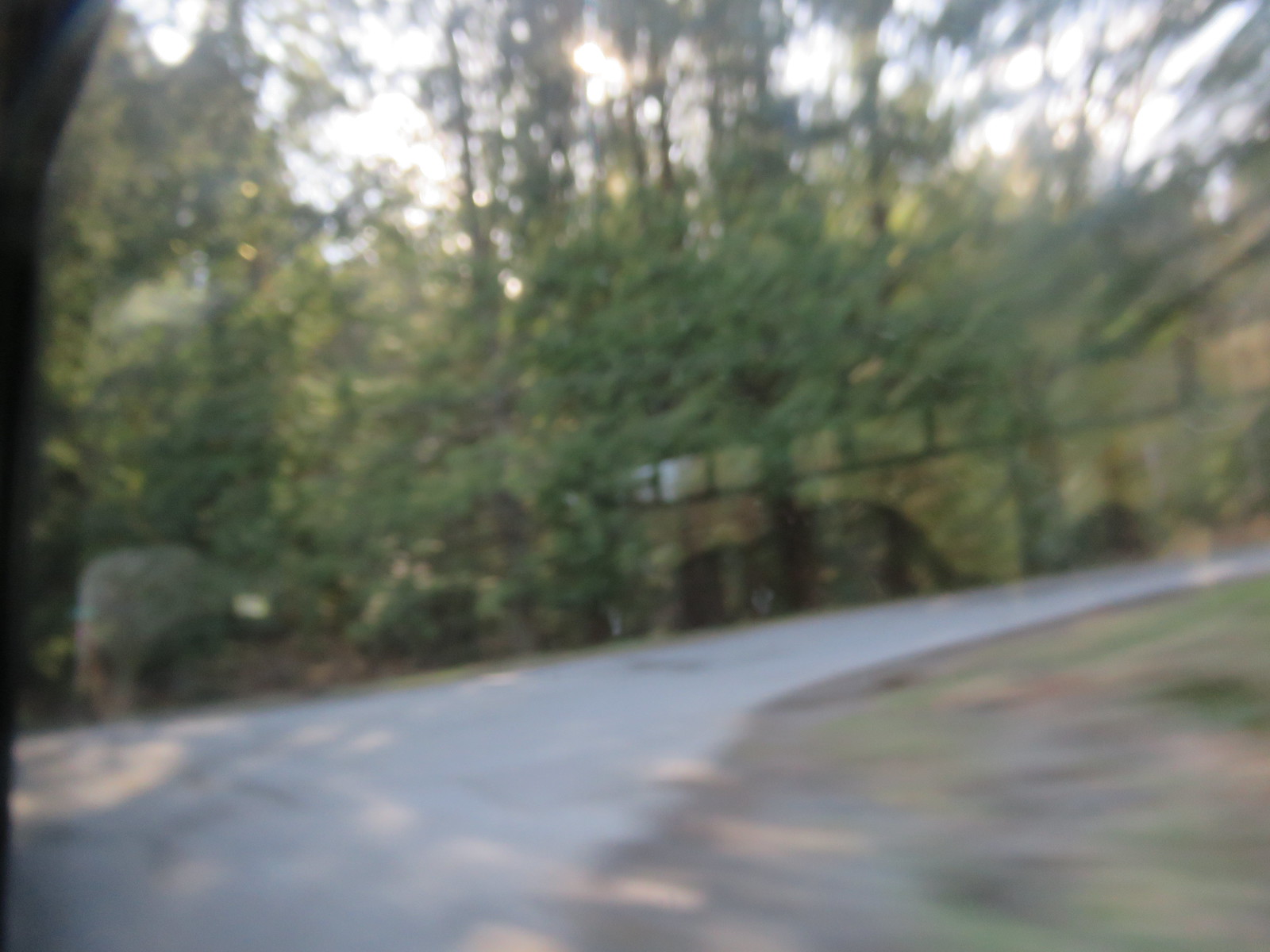This photograph, likely taken from the inside of a moving car, captures an indistinct view through a car window. On the left edge and curving upwards, the dark silhouette of the car's door frame is prominent. The overall image is very blurry and lacks sharp focus. In the background, trees can be seen with sunlight filtering through their branches, adding a faint glow to the scene. Beneath the trees, there appears to be a stone wall, partially obscured by overgrown bushes, although the lack of clarity makes this uncertain. A road runs horizontally across the lower part of the photo without any visible markings. The sunlight, indicative of daytime, enhances the ethereal quality of the blurry landscape.